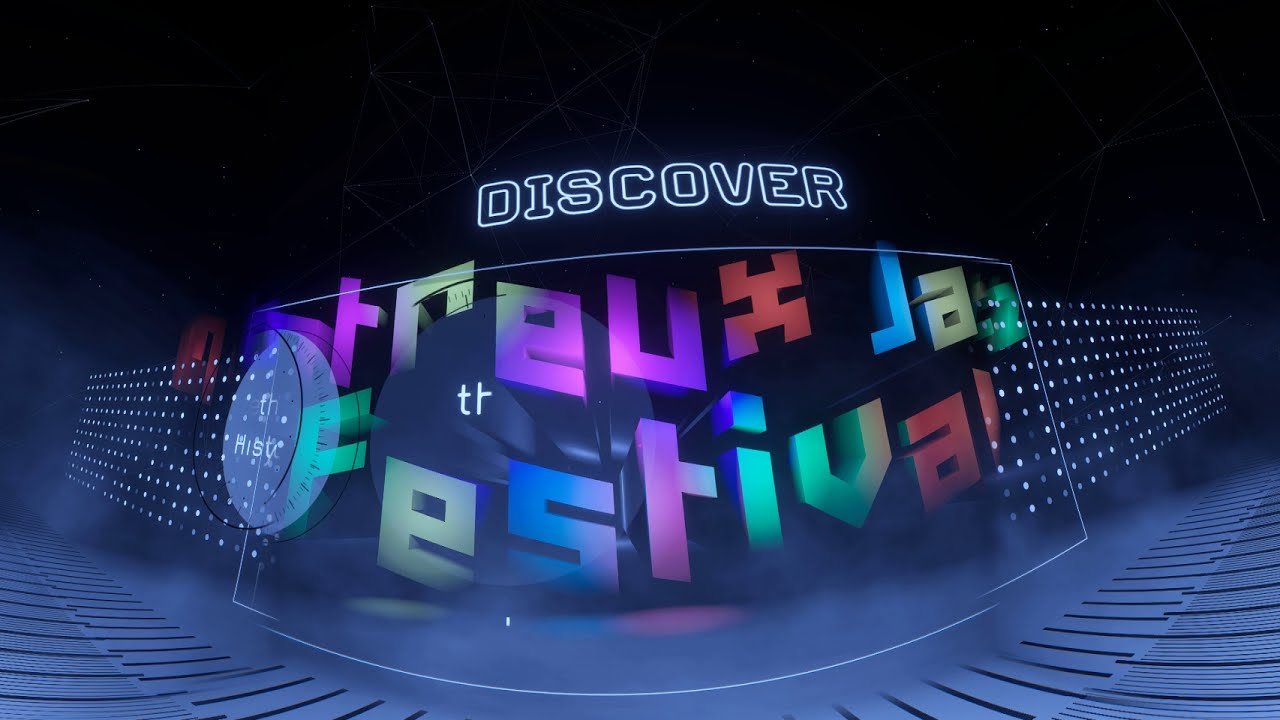This is a vibrant, full-color digital image, likely a 3D rendering, presented in a horizontally rectangular format with no visible border. The top section of the image is dominated by a black background, interspersed with white lines slashing across in varied directions. "DISCOVER" is prominently displayed in neon-like white capital letters, highly visible and futuristic in aesthetic.

Below "DISCOVER," there's an array of computer-generated block letters spelling "MONTREUX JAZZ FESTIVAL," though some letters are hard to distinguish due to the colorful and intricate design. The word FESTIVAL is clearly legible, but the rest of the text, including letters like R, E, U, X, J, A, and even a shape resembling the number 2, adds a complex, almost abstract layer to the sign.

The background remains very dark, accentuating the neon-like colors of the letters which include a palette of pinks, reds, blues, yellows, and greens, creating a striking contrast. Around the text, there are rows of tiny white dots and black slats at the bottom, contributing to a futuristic and dynamic visual. Additional random graphics, resembling headphones and other abstract shapes, are scattered around the letters, enhancing the overall impression that this is a promotional image, likely for an upcoming event such as the Montreux Jazz Festival, known for its international acclaim in the music world.